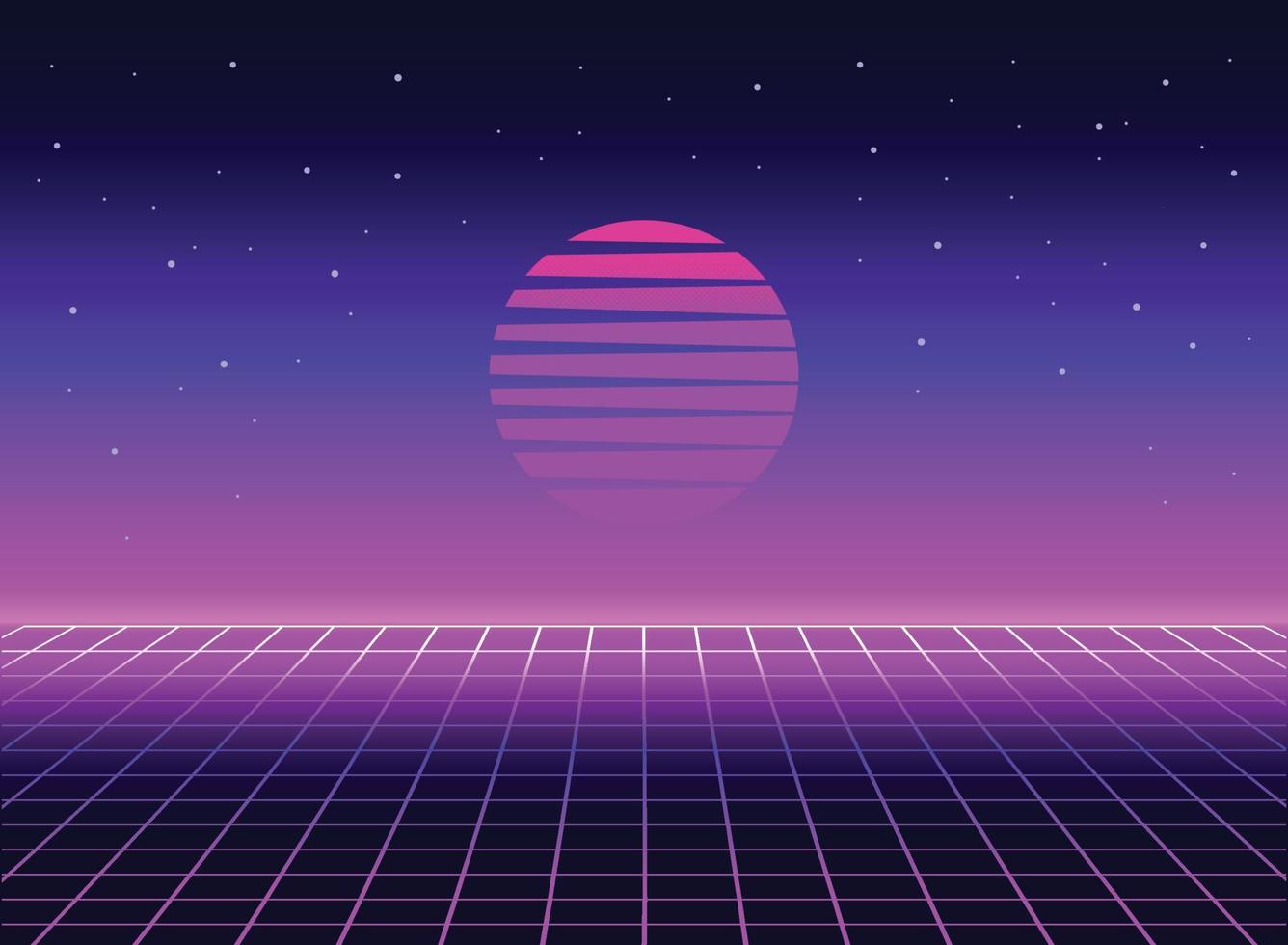The image is a detailed digital creation evoking a disco-style or retro-futuristic aesthetic. It features a dark sky at the top filled with white specks resembling stars scattered across a galaxy. Below this celestial backdrop, the scene transitions into a vibrant, gridded landscape. This grid pattern starts in shades of dark blue at the top, blending into medium purple, lighter blue, and finally into pink hues towards the bottom. The grid lines are primarily pink, blue, and white, creating a checkered tile-like effect across the ground.

At the center of the composition rests a prominent circular shape that appears to be a stylized planet or moon. This circle is pink with horizontal blue stripes, giving it a segmented appearance, as if it's divided into equal horizontal slices. Above this central sphere, the sky once again takes on a darker hue, almost black, heightening the contrast and lending a night-time feel reminiscent of scenes from the classic video game Tron. The overall effect is a striking blend of geometric precision and cosmic wonder, using bold color contrasts and intricate patterns to create a visually captivating digital artwork.